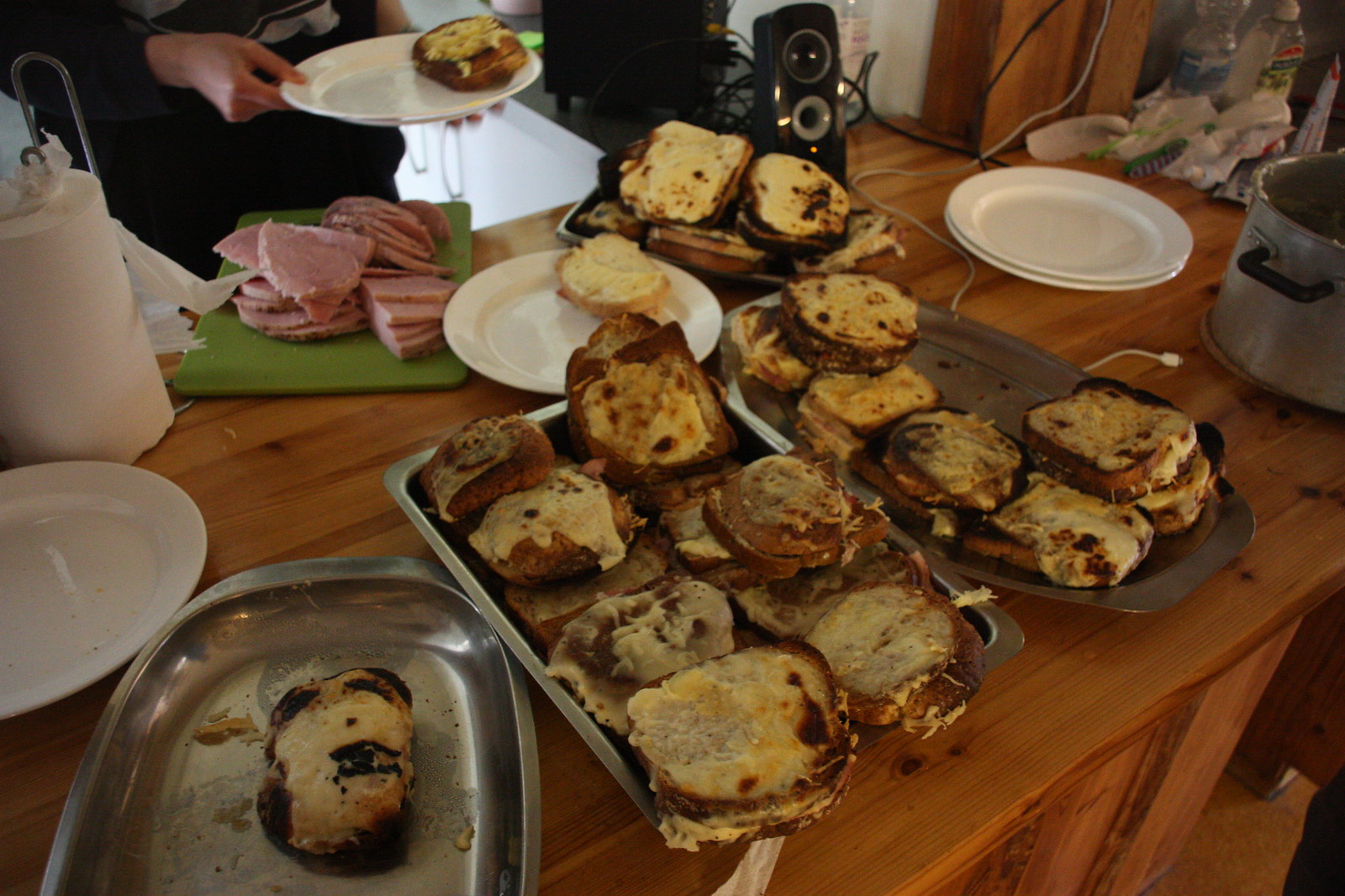This detailed photograph captures an indoor kitchen setting during a casual gathering. At the center of the scene is a large wooden table or counter, adorned with three stainless steel trays of sandwiches. These sandwiches, overflowing with gooey melted cheese, appear to be either grilled cheese or croque monsieur-type sandwiches. Nearby, a green cutting board is piled with thick, pink slices of ham, complementing the cheese-laden sandwiches.

The table holds several other items, including a roll of paper towels and three distinct stacks of white porcelain plates, ready for serving. Additionally, a crock pot and a speaker are visible, adding to the homey atmosphere. In the background, a Caucasian woman in a dark sweatshirt holds a white plate with a sandwich, suggesting that people are helping themselves to the meal.

Overall, the photograph richly conveys the scene of a warm, welcoming homemade buffet, featuring simple yet comforting fare perfect for sharing among friends or family.